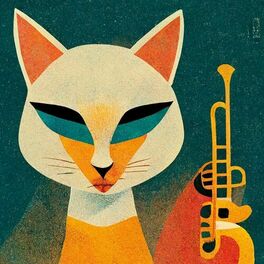This image is a modernist painting of a fox-like cat playing a saxophone, rendered in a distinctive geometric style. The creature features a captivating mix of colors: white intermingled with vibrant fox-orange hues, particularly highlighting its tail. Its compelling turquoise-teal eyes, shaded with a peacock green backdrop, offer a striking focal point, accentuating the animal's unique and expressive personality. The cat's downcast lips and upturned eyes, along with its pointed ears, suggest a moment of interruption, as if it's ready to challenge whoever halted its musical performance. Despite the initial aversion to this style, the cat's intriguing attitude and captivating detail make the artwork resonate in an unexpectedly charming way.